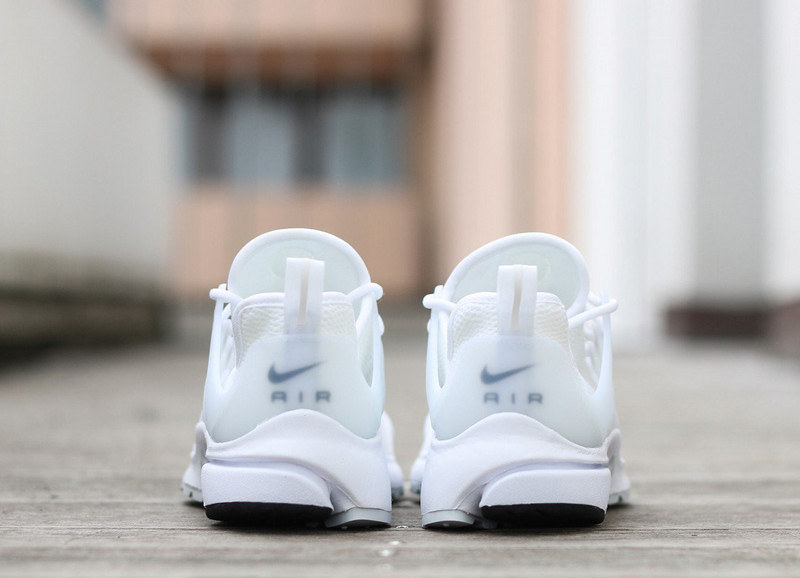Photograph of a pair of high-end, all-white Nike Air sneakers with white shoelaces, placed on a brownish wooden floor outdoors. The shoes are positioned back-to-back, prominently displaying the "Air" logo in gray on each heel with a Nike swoosh above it. The soles are white with black bottoms, featuring a distinct crease around the edge and heel. The background shows a blurry pink-colored building on the middle left and white curtains on the right, adding a hint of surrounding environment while keeping the focus on the shoes.